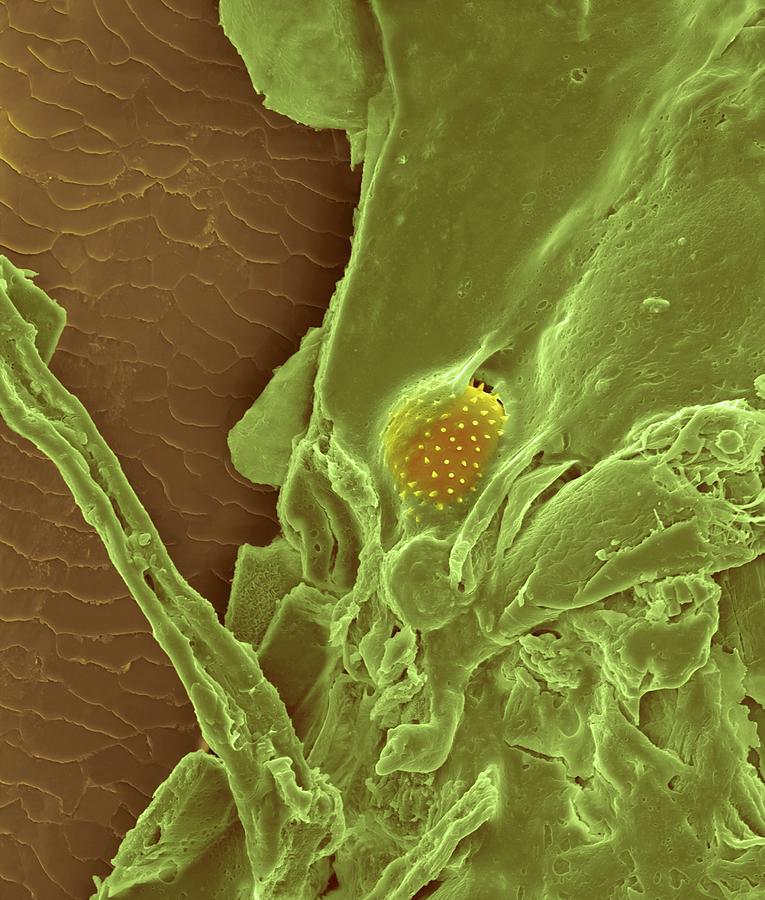The image, likely captured with an electron microscope, displays a highly magnified scene resembling a close-up of skin or another textured surface. On the left side, there is a brown, flaky region that contains ridges and lines, potentially evoking the appearance of skin cells or bark. This area covers approximately one-third of the image. Dominating the right side is a fluorescent, neon green structure that appears almost translucent and spreads across the background. This green substance has a varied texture, with some sections appearing folded or rolled. At the center, slightly off to the left, is a striking yellow, spiky, round object that many compare to a strawberry due to its shape and surface. The yellow object sports numerous little protrusions and sits embedded within the green mass, looking like it might serve a specific function or role. Additionally, emerging from the bottom center and extending to the left are two green stem-like structures, further adding to the textured complexity of the image.